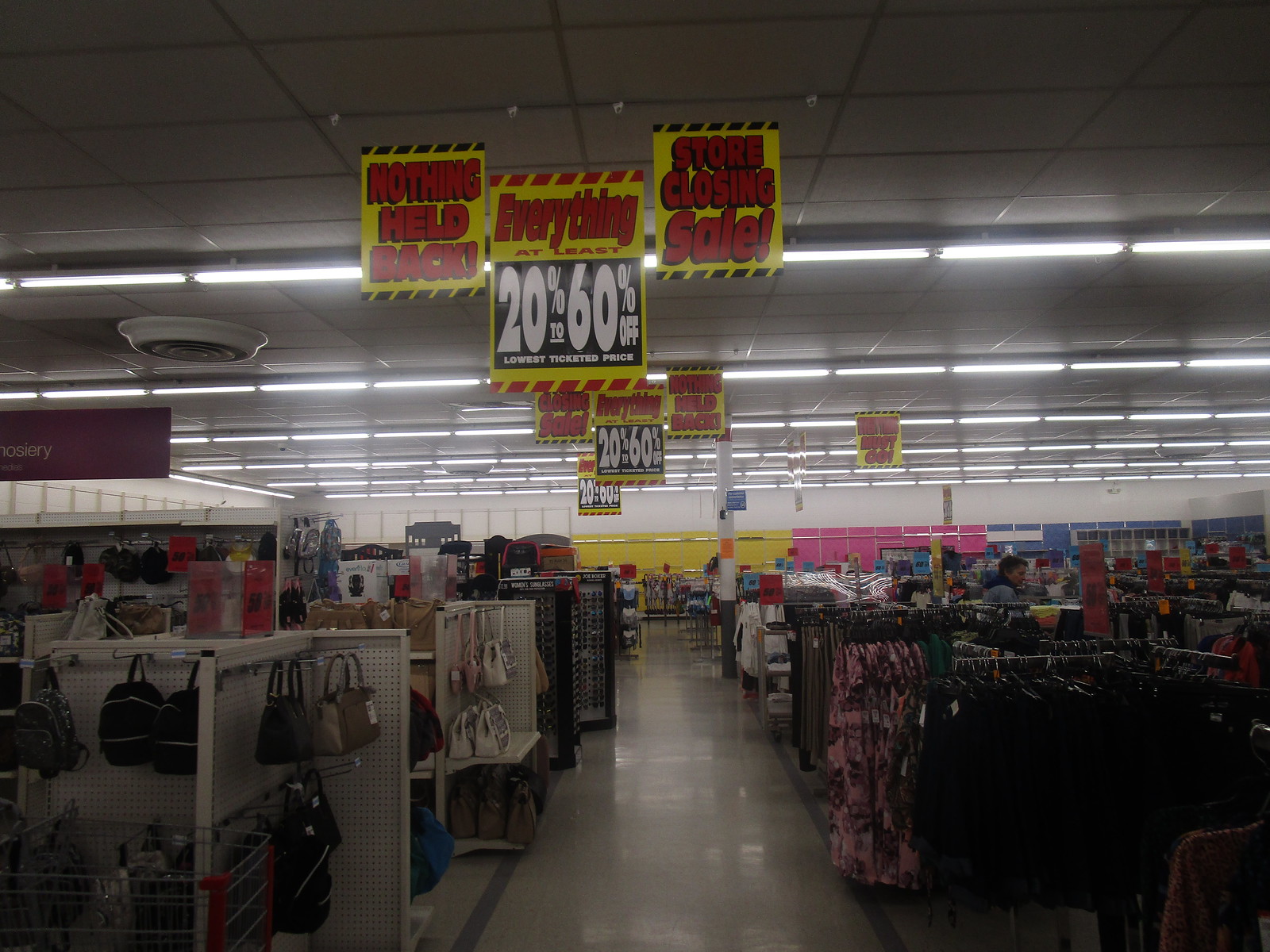This photograph captures the interior of a department store during a store closing sale. The focal point of the image is a glossy, well-maintained pathway that stretches through the foreground. The ceiling above is composed of square tiles interspersed with rows of lights, although the area where the photo was taken appears dimly lit, perhaps due to malfunctioning lights in this specific section.

Suspended along the pathway are vivid yellow signage with bold black borders that reads "Nothing Held Back." Further along, a sign with a red border announces, "Everything 20% to 60% Off," indicating a significant store closing sale in red text. Multiple other signs bearing similar announcements are visible as you continue down the path.

On the right side of the image, rows of individual clothing racks are evident, though the low lighting makes it difficult to discern specific items. It seems either the clothes themselves are dark or the lighting is insufficient in this corner of the store.

To the left, various shelves and racks display an assortment of bags, including backpacks and totes. Moving further down the aisle, one can see stands with sunglasses and their cases. The back wall of the store introduces a splash of color with sections painted in hues of yellow and pink, adding a vibrancy to the otherwise dimly lit scene.